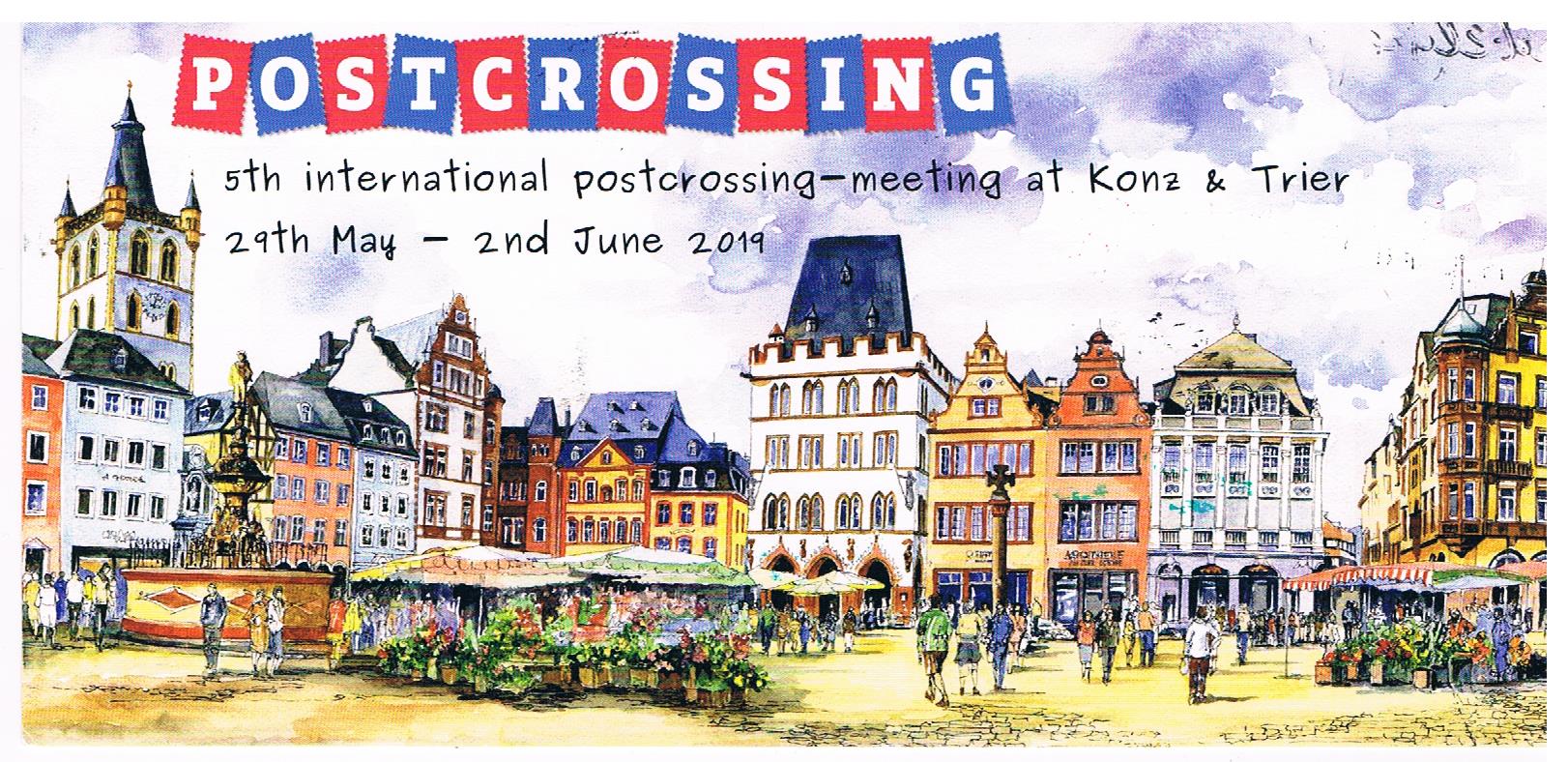The image showcases a beautifully detailed painting of a bustling town center, evoking a European ambiance with its mix of British-like architecture. Numerous buildings, primarily in white, red, and yellow hues with striking blue roofs, stretch from left to right. Prominently featured are flower shops that hint at a lively marketplace, likely akin to a farmers market, with people strolling around the area. On the left side of the painting, a charming fountain can be seen, enhancing the picturesque quality of the scene. The sky above is clear with scattered clouds, all contributing to the vivid illustration.

At the top of the image, the words "Post Crossing" are prominently displayed, with each letter inside alternating red and blue rectangles, and written in white lettering. Below this, the specific event details are clearly indicated: "5th International Post Crossing Meeting at Konz and Trier," scheduled to take place from May 29th to June 2nd, 2019. This detailed painting, possibly intended as a postcard, serves as the notice for the upcoming event.